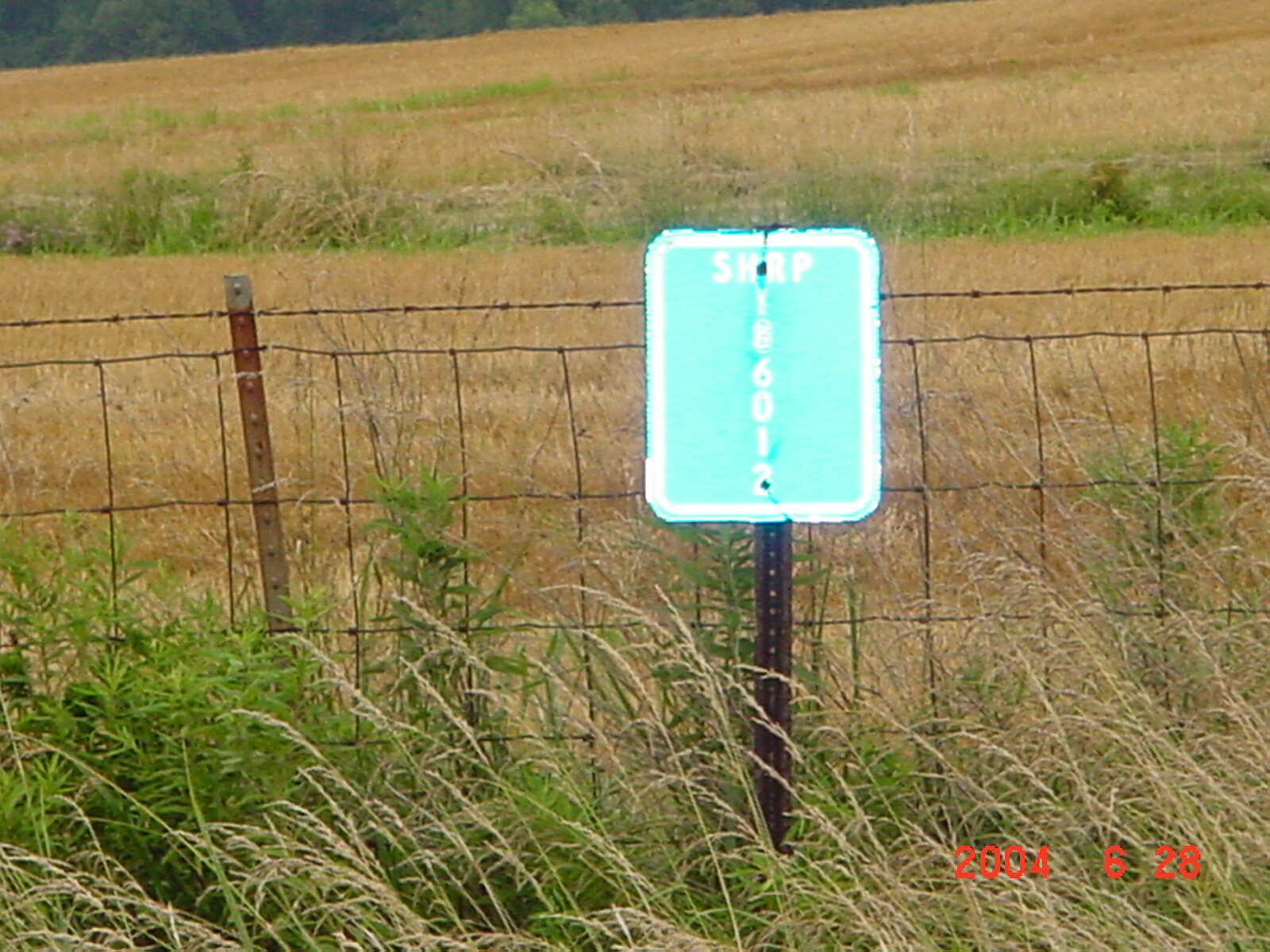The photograph captures a rural scene in the countryside, featuring a field predominantly covered in golden, wheat-like grass with sparse patches of green grass. Among the grass, feathery-topped yellow plants stand out, contributing to the rustic ambiance. In the foreground, a barbed wire fence with brown metal posts delineates the field. A teal-colored sign with white borders is mounted on a post in front of the fence. The sign displays "SHRP" horizontally, and the number "Y86012" vertically beneath it. The background reveals a continuation of the golden grass interspersed with a green strip, likely representing farmland. A date stamp in the bottom right corner reads June 28, 2004.